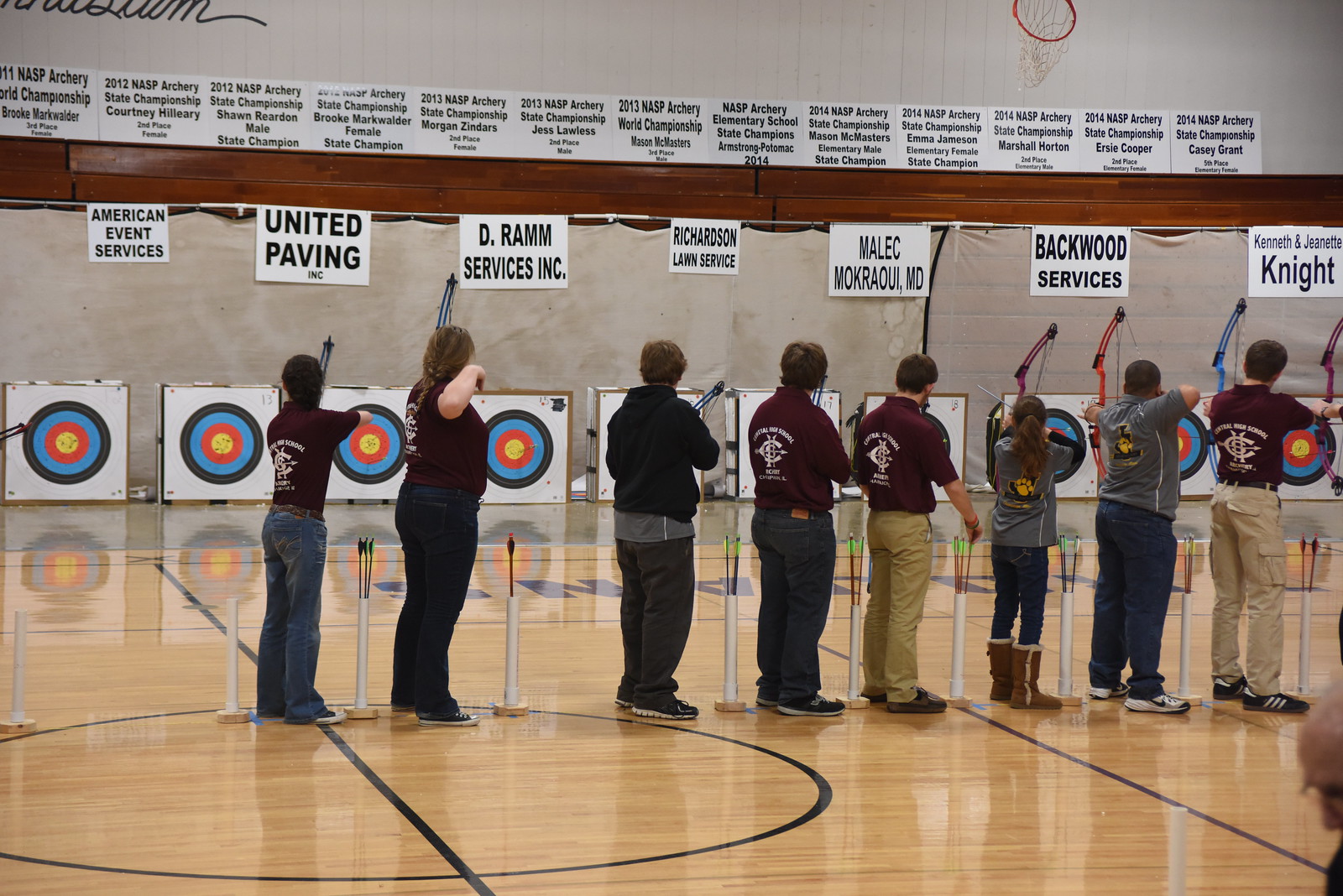This photo captures an indoor archery event taking place inside a basketball court. The scene features eight or possibly more young competitors, both male and female, lined up against the wall, each equipped with a quiver of arrows and various colored bows, including burgundy, red, and blue. Each archer is positioned in front of their own target, which are white with concentric circles in black, blue, red, and a yellow bullseye. The upper portions of the wall are adorned with signs celebrating past NASP Archery state and world champions, like Courtney Hillary and Shawn Reed, among others, showcasing their accolades from different years and competitions. Below these championship banners, another set of signs displays the names of sponsors supporting the event, including American Event Services, United Paving Incorporated, DRAMS Services Incorporated, Richardson Law Service, and Malik, Moravow MD, among others. The image captures a vibrant and focused atmosphere of youthful determination and community support.